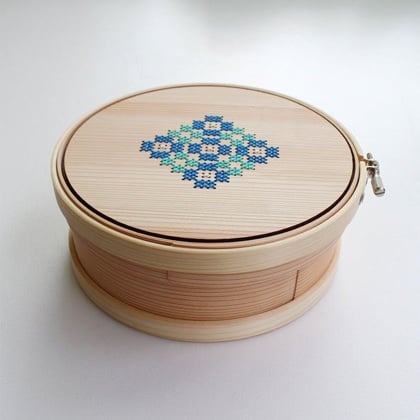The photograph, taken indoors, showcases a unique drum-shaped wooden storage box prominently in the center, silhouetted against a white to light gray backdrop. This light tan, wooden container bears resemblance to a sewing implement but appears to deviate from typical designs. The lid is adorned with a series of alternating blue and green stitches, crafted into a checker pattern forming a larger square, which is intricately embroidered directly onto the wood rather than cloth—a rare needlepoint technique. To the right side of the box, a small padlock secures the lid through two metal hoops, one on the base and one on the top, emphasizing its functional yet decorative nature. The detailed stitching and the drum-like structure, complete with a wooden tightening band, add to the uniqueness of this piece, casting a shadow towards the bottom left hinting at the light source from the opposite side.